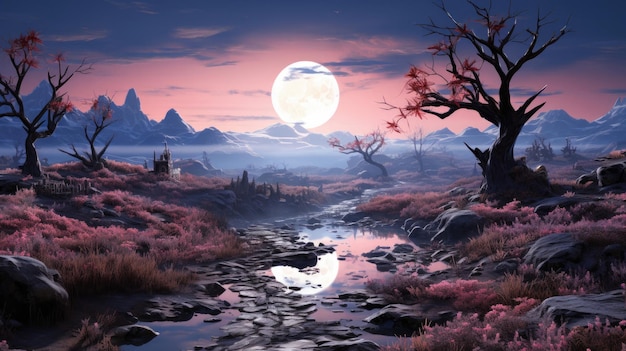This illustration, seemingly computer-generated or AI-created, presents a fantastical and moody landscape. Dominating the scene is a vibrant but eerie color palette of pinks, purples, and blues. At the center, a winding stream reflects a massive full moon and the surreal sunset-like colors of the sky, casting a haunting glow. The sky is adorned with dark, wispy clouds and is primarily a mix of pink and purple hues.

On either side of the stream, the landscape is dotted with jagged boulders and gnarled trees, most of which are nearly bare with occasional red and orange leaves clinging to the stark branches. Some of the smaller trees and foliage display varying shades of pinks and reddish oranges, contributing to the otherworldly ambiance. The grass surrounding the river ranges in color from reddish-pink to purple, providing a surreal contrast to the natural elements.

On the horizon, sharp, dark gray and bluish mountains rise on both sides, framing the enormous moon that seems to hover just above them. Gray mist permeates the scene, adding to the ethereal quality of the artwork. The nearly dry creek bed in the foreground shows patches of water that mirror the moon and sky, emphasizing the reflective and mesmerizing elements of the illustration. Overall, the image exudes a fantastical, almost fairy-tale-like atmosphere, where the boundary between reality and fantasy is delightfully blurred.